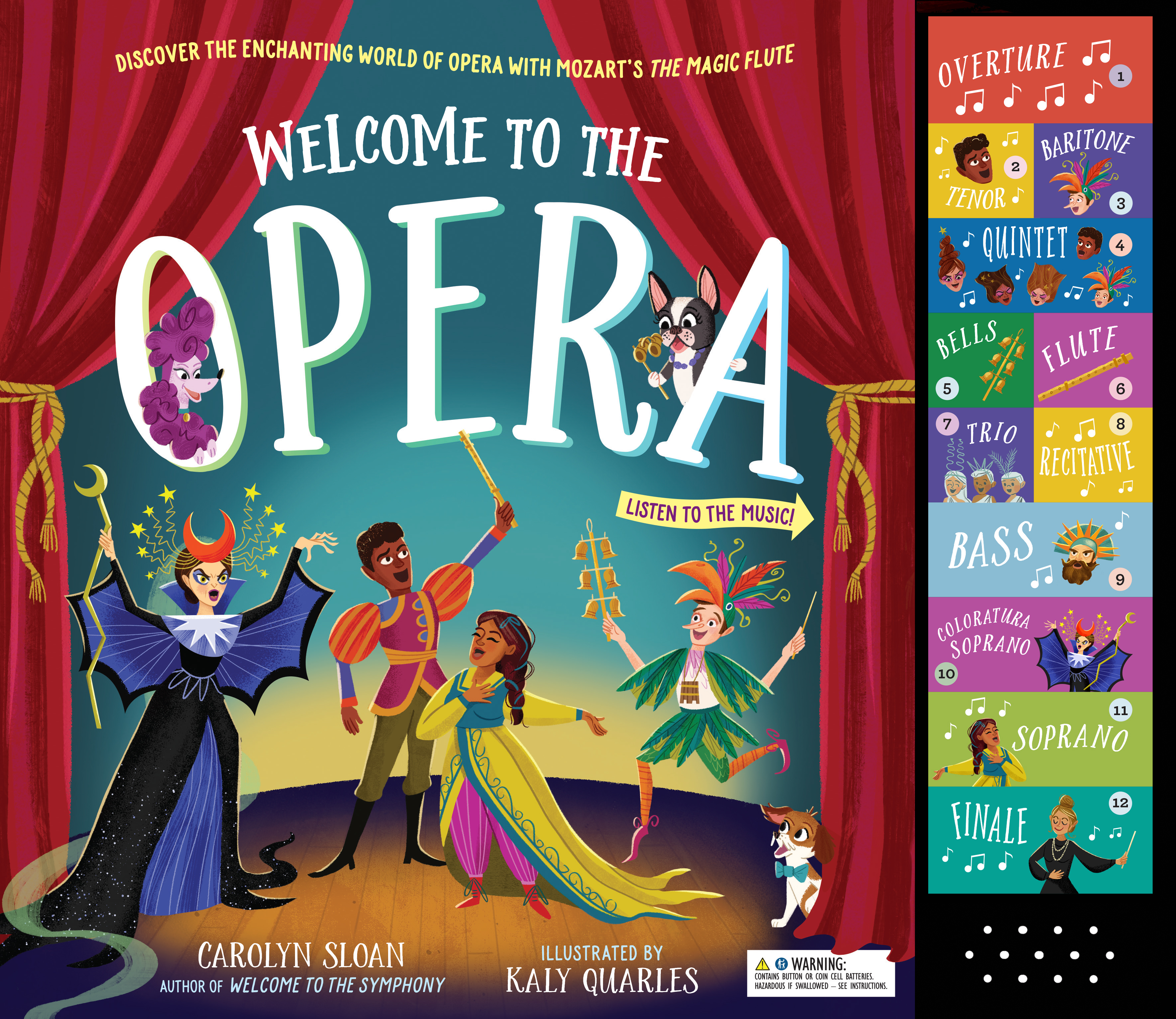**Album Cover: "Discover the Enchanting World of Opera with Mozart's The Magic Flute"**

This vibrant cartoon-style album cover is a visual celebration of Mozart's opera "The Magic Flute." On the left-hand side, a stage adorned with elegant red curtains tied back with golden ropes welcomes viewers with a large white-font inscription: "Welcome to the Opera." Above this welcoming message, in an enchanting script, it reads, "Discover the enchanting world of opera with Mozart's The Magic Flute."

Beneath these inviting words, a vivid scene unfolds. A witch, cloaked in purple and black with dramatic bat-like sleeves and devilish horns, brandishes a magic wand, embodying an air of mystique. Next to her stands a singing prince, harmonizing with a princess dressed in an ornate Middle Eastern costume reminiscent of Princess Jasmine, complete with balloon-style pants that accentuate her regal charm. Adding a touch of whimsy, a jovial court jester, adorned with a traditional multi-pointed cap and jingling bells on a stick, entertains. Scattered throughout this fanciful tableau are various dogs, adding a playful element to the scene.

On the right side of the cover, nestled within colorful squares that segment the different parts of the opera, is a detailed breakdown of the musical components. Each square, with its distinct hue and character illustration, corresponds to a specific part of the opera, numbered 1 through 12. The segments are labeled as follows: Overture, Tenor, Baritone, Quintet, Bells, Flute, Trio, Recitative, Bass, Coloratura, Soprano, and Finale. In each box, characters sing their respective parts, encapsulating the rich and dynamic range of Mozart's composition.